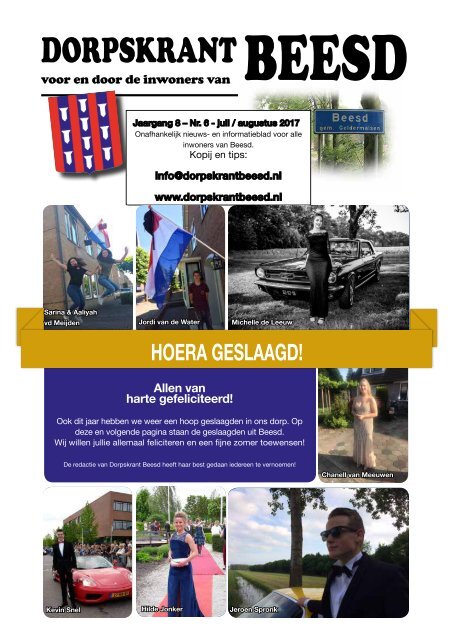The image is a detailed poster or front page of a newspaper, likely from the Netherlands, titled "Dorpskrant Meester." The text below the title says "Voor en door de inwoners van," indicating it is for and by the residents. It features a date from 2017 and a website address, www.dorpskrantpied.nl. The main content includes several well-positioned images: at the top right is a street sign, in the center are people, including girls playing outside near a building, and a girl standing in front of a car. At the bottom, a well-dressed man stands next to a sports car. Additional images show people jumping, a person beneath a Dutch flag, and a black and white photo of a woman in front of an American car. The text, all in Dutch, includes phrases like "Village Newspaper," "Volume number 8," "January to August," and "independent news and information for all residents." The colors in the image are predominantly white, black, red, purple, gold, pink, blue, brown, gray, and yellow. The setting appears to be an advertisement or poster for a community event or competition, with names of contest winners and several subheadings in blue and white text.